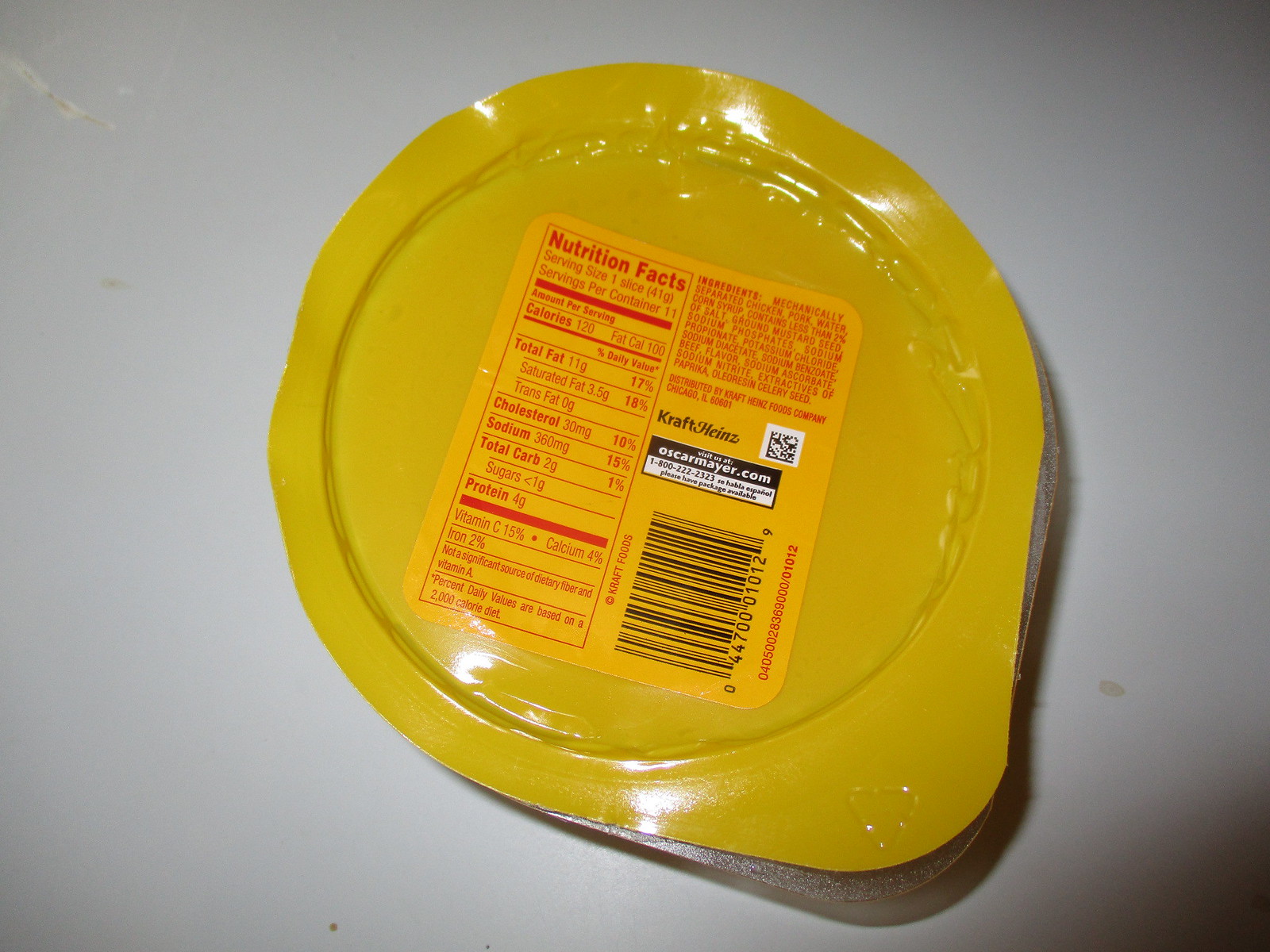This image captures the back label of a packaged cold cut product produced by Oscar Mayer, a brand under Kraft Heinz. The photograph presents an overhead view focusing on the yellow label situated at the bottom of the packaging, thus obscuring the meat itself from view. The label prominently displays nutritional information: each slice contains 120 calories, with 100 of those calories deriving from fat. Breakdown highlights include 11 grams of total fat, 3.5 grams of saturated fat, 10% of the daily recommended cholesterol (30 milligrams), a significant sodium content, minimal carbohydrates, and a generally high fat composition. The ingredient list leads with mechanically separated chicken, pork, water, and corn syrup, although the specific type of meat remains unspecified. This detailed label hints at a product that is notably high in fat content.